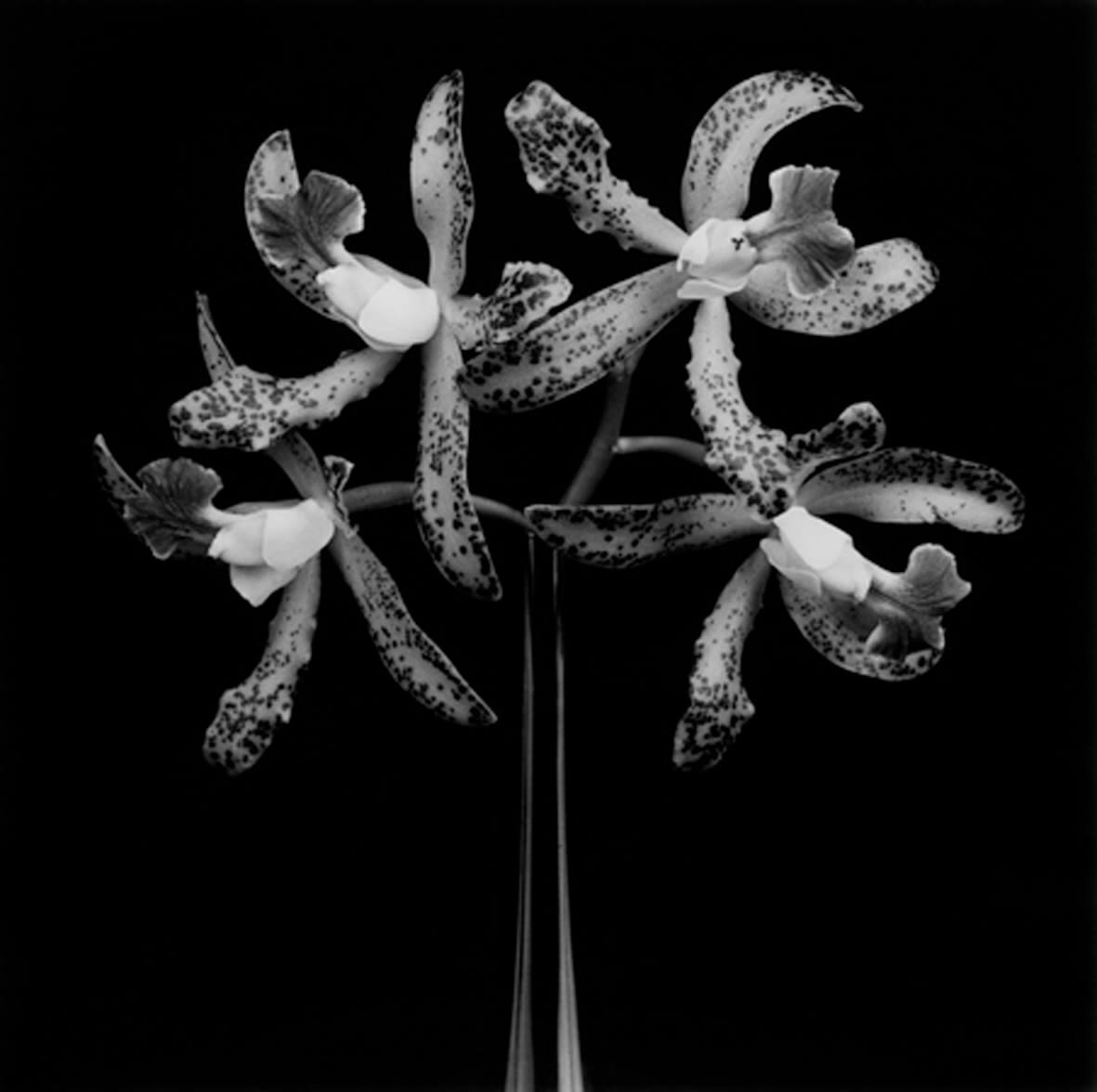This striking black and white photograph features a dark, solid black background that accentuates the main subject: four starfish-shaped flowers. The flowers are prominently centered in the frame, growing from a single stalk with slim, elongated leaves. Each flower has five petals adorned with black speckles, creating a stark contrast to their white petals and gray-toned stems. The blooms exhibit a lily-like shape and are fully opened, with central buds clearly visible. Two of the flowers directly face the camera, while the other two are angled towards the left and right, adding a dynamic balance to the composition. These flowers occupy most of the upper two-thirds of the image, emerging from a clear vase at the bottom, making for a modern and elegant visual presentation.